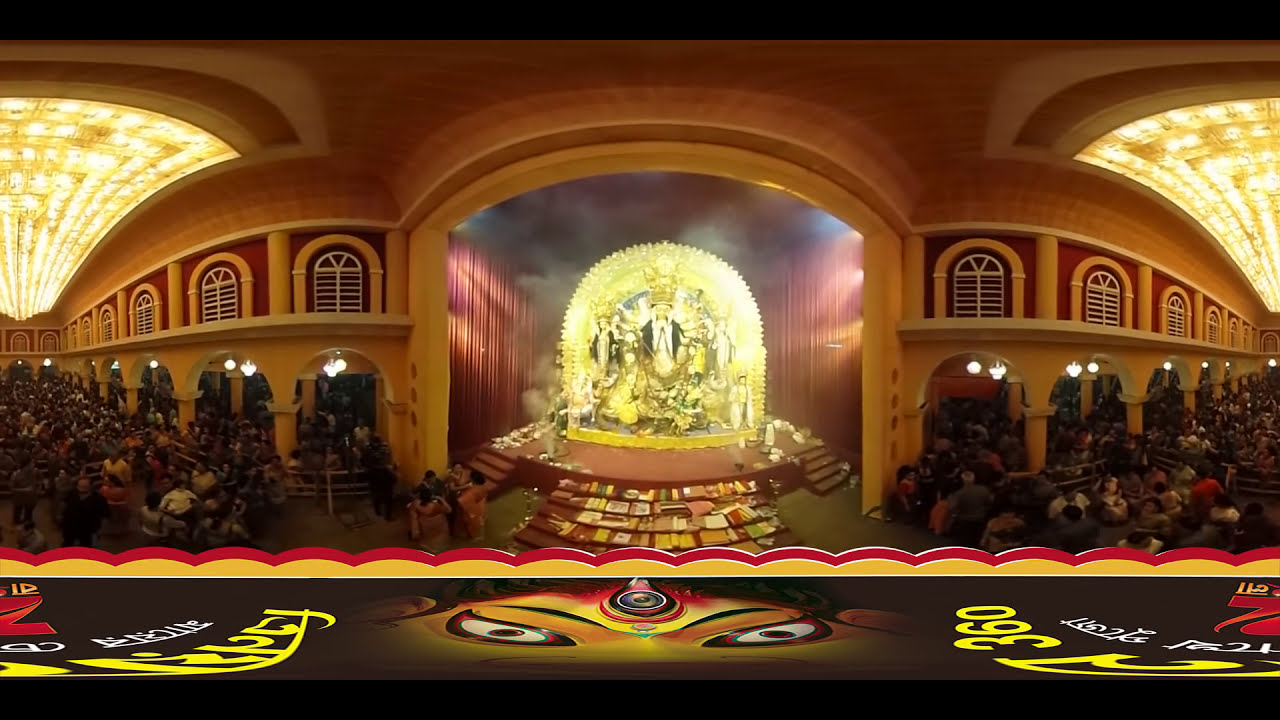The wide rectangular panoramic image, bordered at the top and bottom by thin black rectangles, depicts a vibrant and distorted indoor scene resembling the interior of a grand house of worship or a festive hall. Central to the composition is a glowing, golden shrine or statue, crowned by a vivid yellow display, standing on a theater deck with a red bottom. This central structure is flanked by walls with maroon hanging curtains extending into the background, which curve and arch upwards, enhancing the sense of grandeur.

Immediately below the shrine, a startlingly vivid artwork spans across the image, featuring a yellow character with striking white and red eyes, framed by red and black designs, and bordered by yellow and red. The artwork includes yellow and white text in another language on both sides, though the text is mostly indecipherable save for the number “360” on the right.

The setting is bustling with large groups of people on both the left and right, positioned within an elaborate interior of yellow walls adorned with red designs and golden ceilings. The upper portions of the structure feature brown archways separated by columns, with arches decorated by door decals and illuminated by lights hanging from their tops. Below these elements, the walls give way to a lighter gray level before transitioning back to brown arches at the bottom, each one adorned with hanging lights.

The distorted lower section of the image reveals a curious central motif: two discernible eyeballs within a metallic-colored circle, framed by eyebrows and additional hues of yellow and red. The setting, resplendent with colors including black, brown, gold, purple, blue, red, green, and yellow, evokes a festive atmosphere heightened by the visual distortion, drawing the viewer into a captivating, almost surreal spectacle.